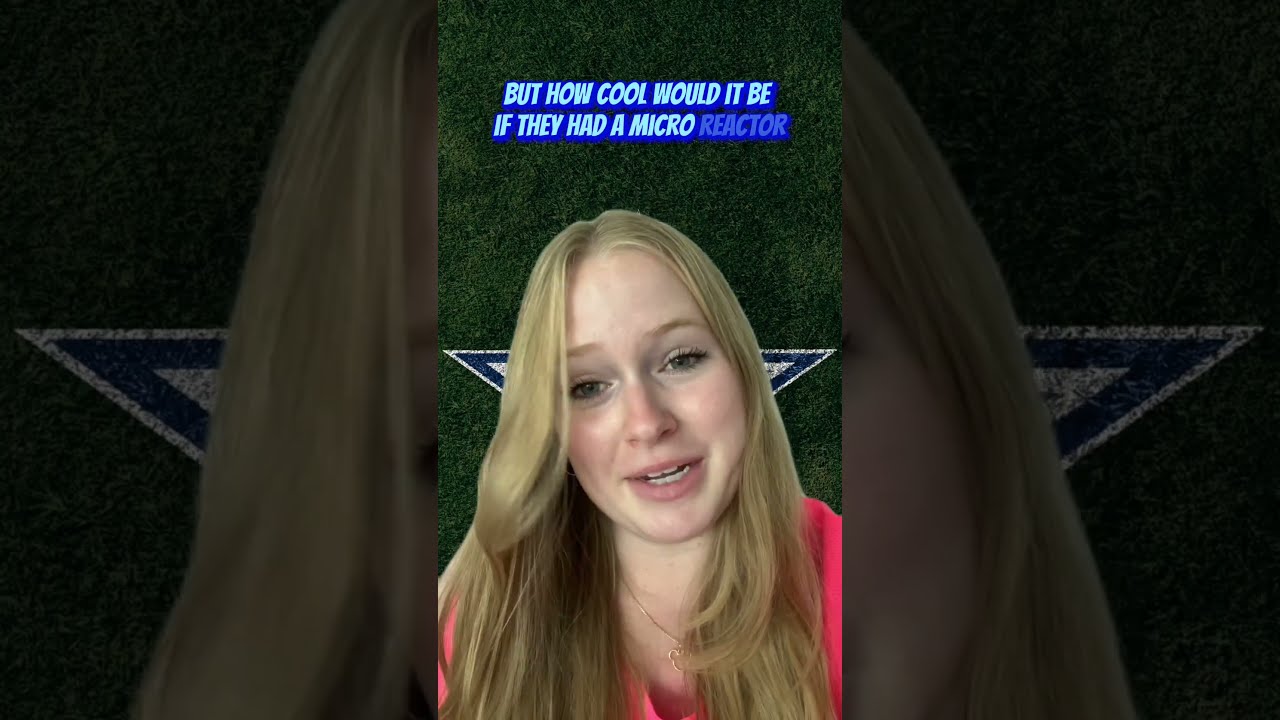The image is a horizontally-oriented composite photograph featuring a young blonde woman as the central subject. She has long, flowing blonde hair and is wearing a pink shirt paired with a silver necklace adorned with a small, golden Mickey Mouse head. Her eyebrows are thin and blonde, and she has pink lips.

The background of the image is predominantly dark, showcasing astroturf on either side, resembling a football field, specifically hinting at the Dallas Cowboys due to the visible white and blue triangles resembling points of the iconic Cowboys star logo.

Above the woman’s head, there is a bold, white, all-caps text with a deep blue shadow that reads, “BUT HOW COOL WOULD IT BE IF THEY HAD A MICRO REACTOR?” Additionally, blue arrows or small triangular shapes near her head create an illusion that makes her ears appear pointed. The composition seems to integrate another darker image of the back of her head into the background, enhancing the layered, composite effect of the photograph.